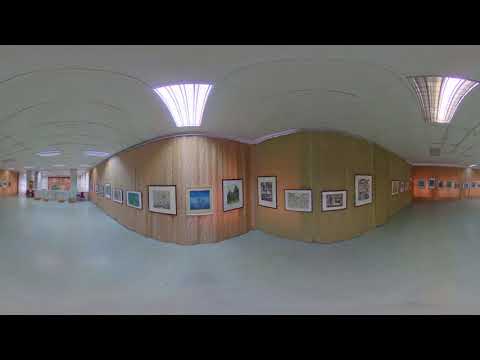This is an interior panoramic shot of a building that resembles an art gallery or museum. The room features a plain gray stone floor and a white paneled ceiling adorned with rectangular lights. The walls are covered in vertical wooden slats, creating a warm and inviting atmosphere. Lining these wooden walls are several framed pictures or artwork, each enclosed in a brown frame with a thick white border. The frames, which vary in size from rectangular to square, stretch from the center left to the far right of the image. To the left of the room, there is a counter area, also set against a background of wood paneling. The overall perspective of the image is slightly distorted, giving the appearance of the walls curving inward in the middle before straightening out again.